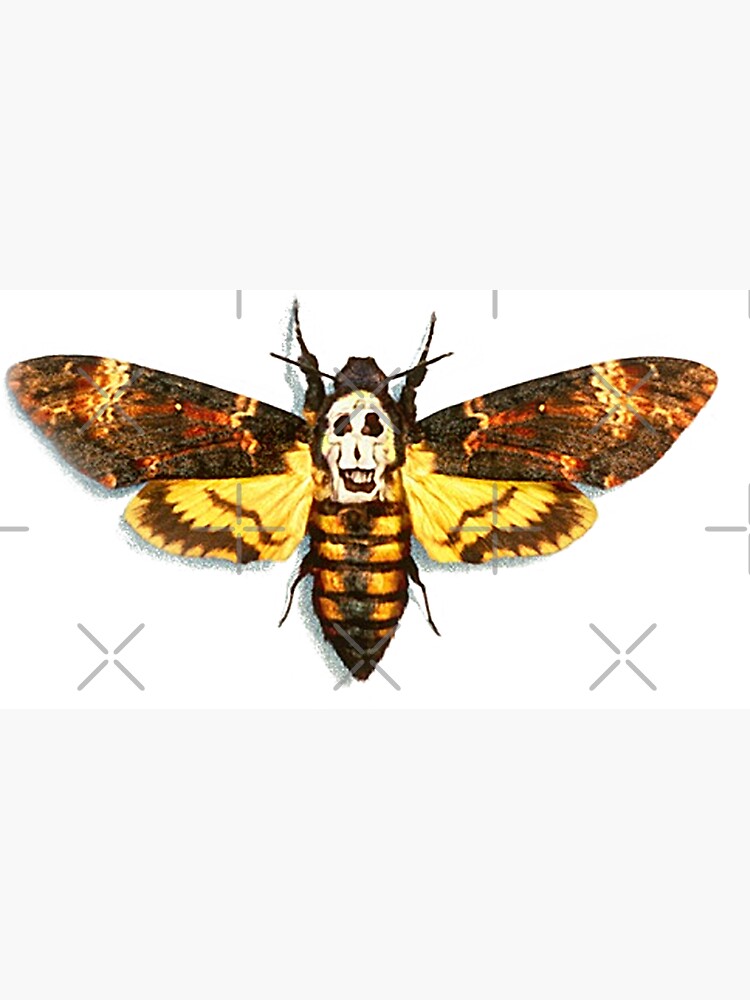This image features a moth with a distinctive design and detailed features. The overall composition is rectangular, with the top portion displaying off-white to white shades, transitioning to a central area that is entirely white adorned with gray dotted X's. The focus of the image is a brown and tan-colored moth, characterized by a thick body with black, brown, and tan stripes, resembling a bee's body, and four visible legs—two at the top and two at the bottom. The moth's wings are predominantly yellow with brown trim and patches of gold, brown, and orange, showcasing a beautiful array of colors. Notably, the moth's back bears a striking design that resembles a white skull with black eyes and a mouth, creating an eerie but fascinating visual effect. The moth's head features two prominent antennas, adding to the intricate details of this captivating insect.